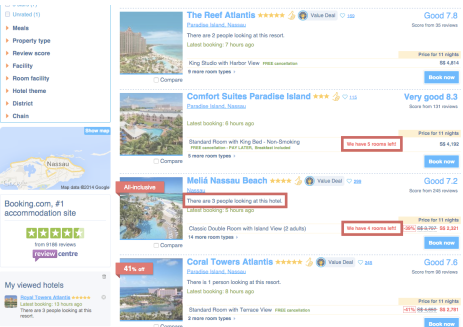A detailed screenshot captured from Booking.com, showcasing an accommodation search page. The interface features a predominantly white background, with a left-hand column dedicated to various search filters like property type, number of rooms, and more, though the text appears quite small and hard to decipher. Below these filters is an integrated map displaying the search area, followed by Booking.com's statistical ratings indicating the site's reliability.

On the right side, which occupies the majority of the screenshot, four search results are presented. Each result includes a square thumbnail image representing the property, accompanied by the accommodation name highlighted in blue. Directly below the name, additional information is provided, such as pricing details and booking options. Each listing also features a user rating indicated by terms like "Good" or "Very Good" in the top-right corner. Notably, two properties have a special offer indicated by a red box. Further, the person who took the screenshot has highlighted certain information with red blocks, drawing extra attention to those details.